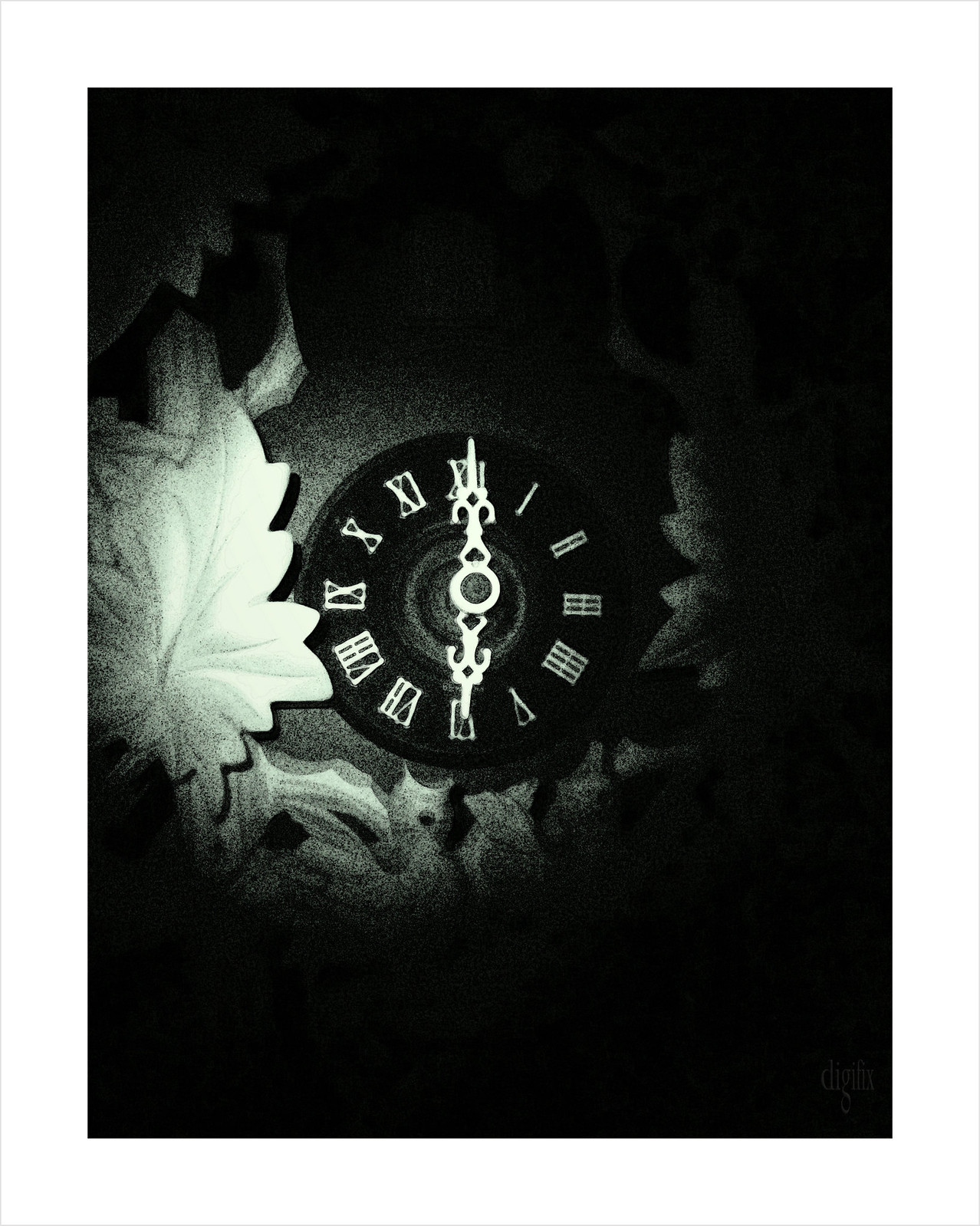In this grainy, black-and-white image reminiscent of night vision photography, a central illuminated clock draws immediate attention amidst an expanse of dark shadows. The clock, round and affixed to a wall, features a dark — likely black — face adorned with white Roman numerals. The time displayed is approximately 6 o'clock. Surrounding the clock are large, decorative leaf decals extending outward from the center, with the left side more illuminated, offering a clearer view of the intricate details. The contrast between the illuminated center and the shadowy periphery creates a dramatic focal point, emphasizing the ornate clock and its surrounding adornments.